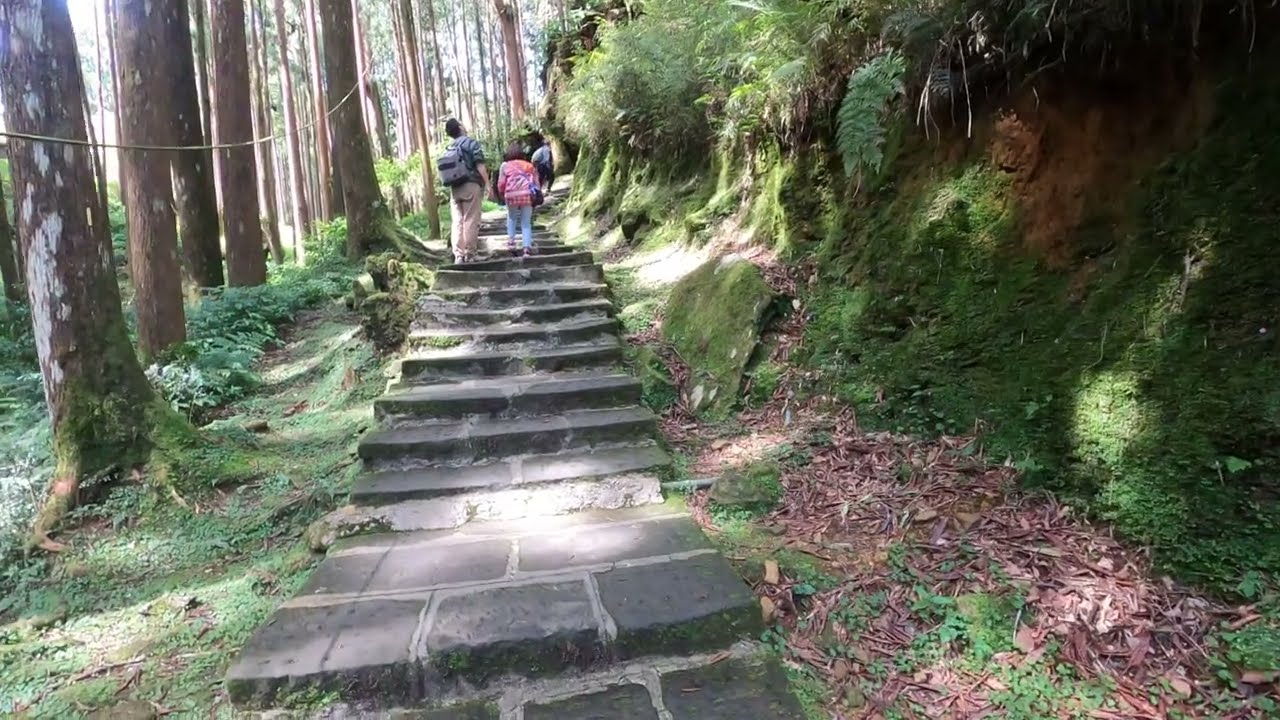The image depicts a serene forest path, paved with a series of stone bricks that form steps leading up a hillside. The path starts at the bottom center of the picture and extends towards the top, framed by rich green vegetation peppered with brown patches of wood shavings and fallen leaves. To the left, several old trees stand tall, their trunks adorned with white speckles, and a rope barrier runs alongside them. In the center of the path, multiple people are seen walking. On the left is a man clad in tan pants, a blue shirt, and a gray backpack. Next to him on the right, a woman wears blue jeans and a pink sweater, carrying a brown purse. Off in the distance, another hiker can be spotted further along the path. The lush, moss-covered hillside flanks the right side of the trail, adding to the natural beauty of the scene.